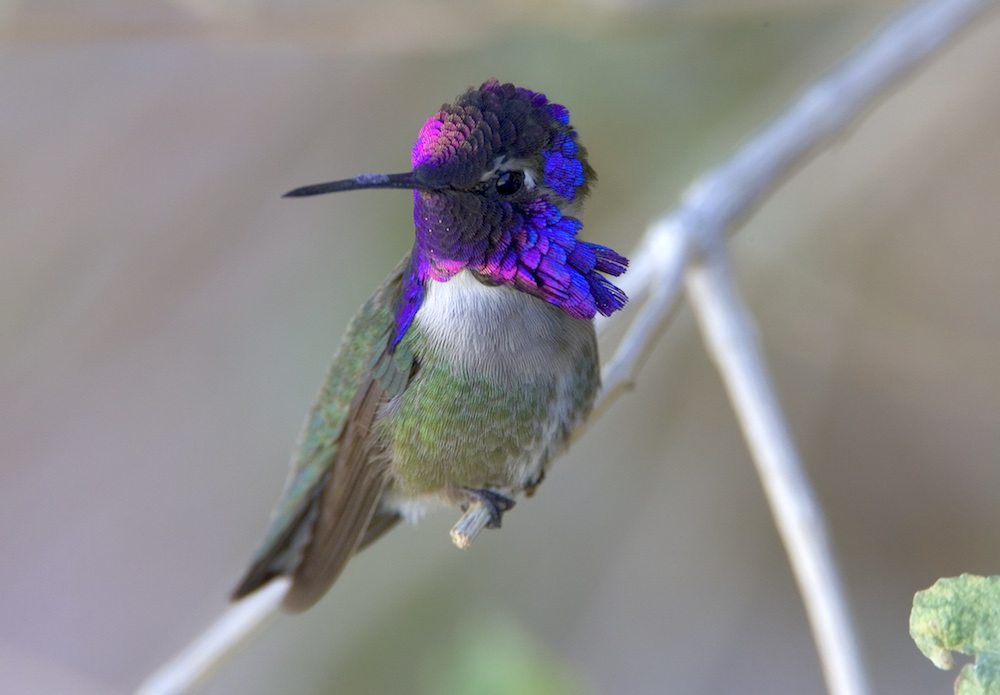The image is a close-up photograph of a stunningly colorful hummingbird perched on a delicate, twig-like white branch, which angles to form an upside-down Y shape. The hummingbird's head is turned to the left, showcasing its brilliant, almost neon feathers that are a striking mix of magenta, blue, and purple. Its slim, long beak is predominantly black with a distinctive spot of blue, and it stands out against its one visible dark eye. The bird's chest is white, transitioning to a vibrant green as it extends downward toward its body and wings—where the wing feathers show hints of greenish-yellow with brown underwings. The background is muted and blurred, predominantly shades of green and gray, providing a soft backdrop that makes the bird’s vivid colors pop. One green leaf peeks out in the bottom right corner, adding a subtle touch of natural context to the beautifully detailed image.